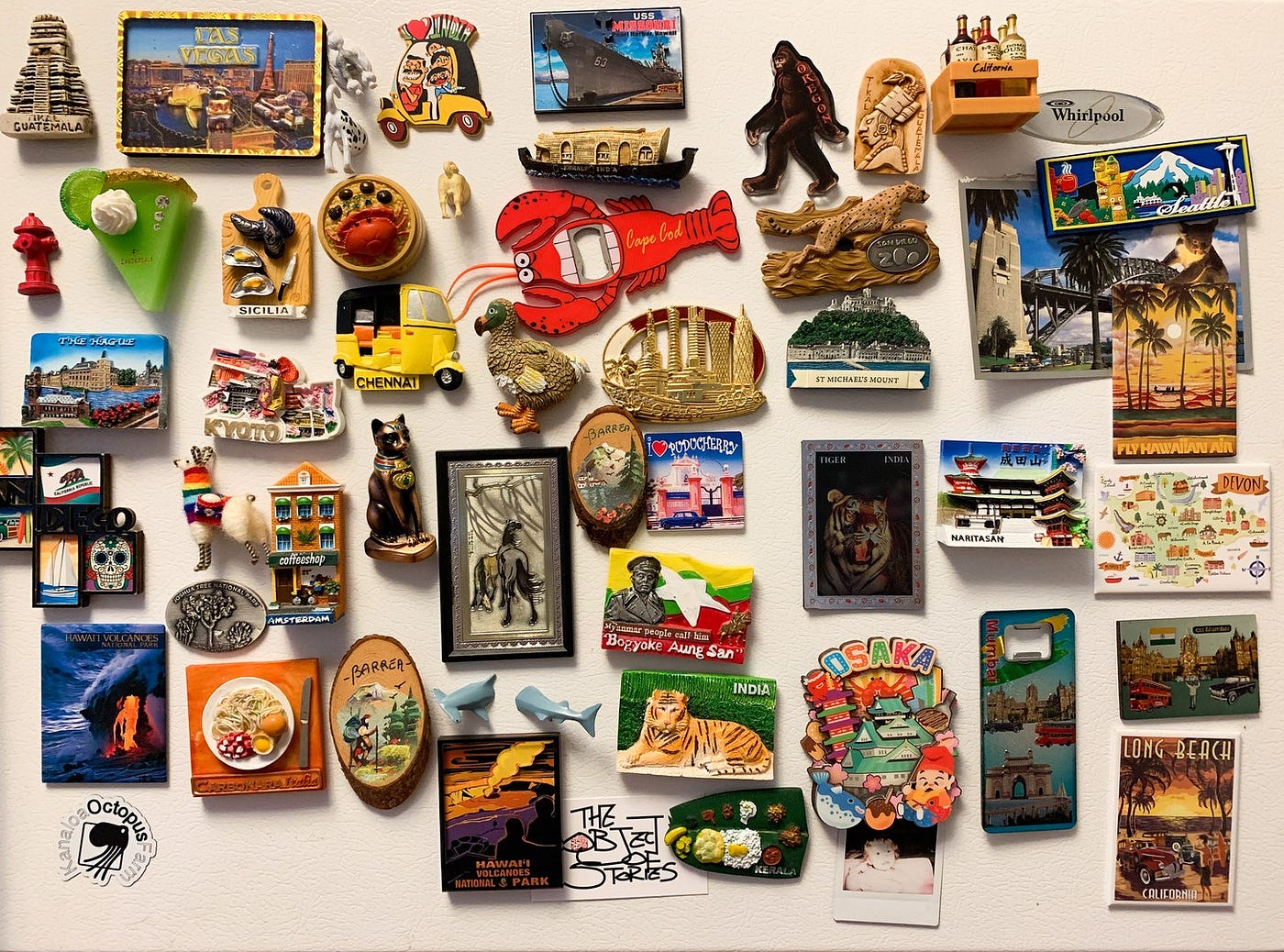The image is a detailed photograph of a white refrigerator surface covered with an eclectic assortment of novelty magnets, mostly of varied shapes and sizes often collected from tourist destinations. The magnets are arranged haphazardly, spanning the entire surface from the top left to the bottom right corner. The assortment includes colorful representations such as a big red cartoon lobster, a novelty can opener from Cape Cod, a yellow tuk-tuk labeled "Chennai," and a vibrant orange and black striped tiger inscribed with "India." Other notable magnets depict a palm tree scene with "Fly Hawaii," a blue shark, a King Kong on ice skates, a shelf of wine bottles, an engraving of a medieval Japanese castle, and a magnet labeled "Long Beach." Despite the tiny text on the magnets being unreadable, the array features a diverse palette with colors like yellow, black, red, white, multiple shades of green, purple, orange, and various blues, giving the fridge a vibrant, travel-memento-adorned appearance.